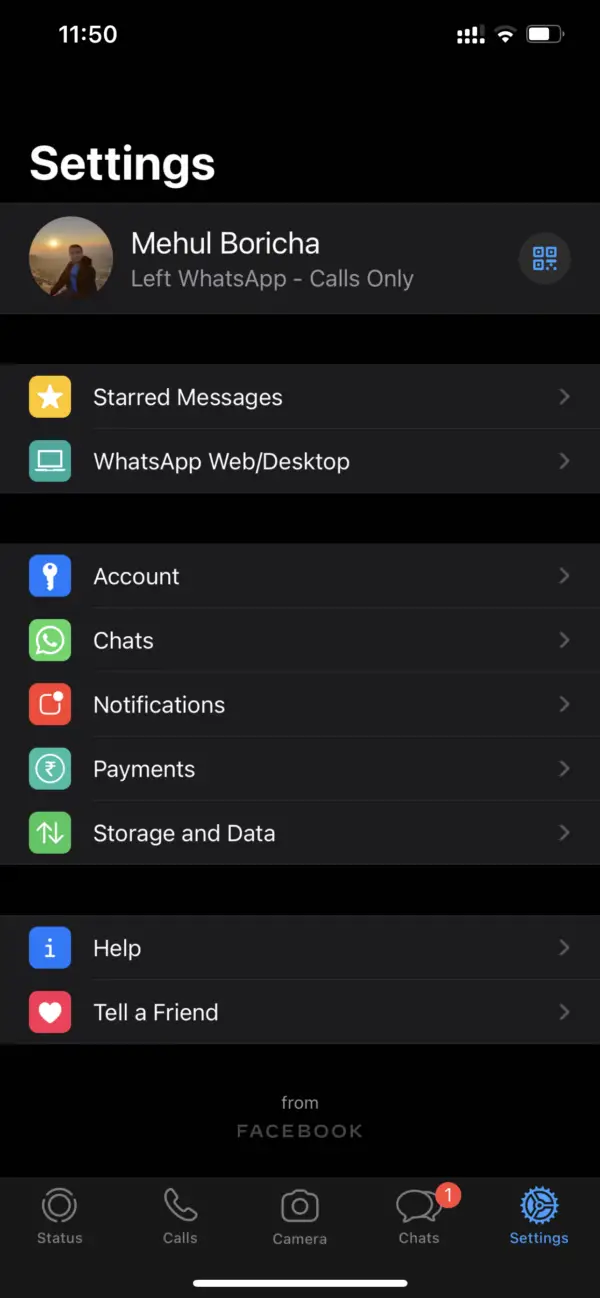A detailed screenshot of a cell phone screen displays the "Settings" menu of the WhatsApp application. The top-left corner shows the current time as 11:50. In the top-right corner, various status icons are visible, including the cell phone reception, Wi-Fi signal strength, and battery level indicator. Dominating the upper section of the screen, the word "Settings" is prominently displayed in large white font.

Directly below the "Settings" heading, there's a circular profile picture of a man, captured against a backdrop that resembles a sunset. To the right of the profile picture, the text reads "Mehul Boricha" with the subtitle, "Left WhatsApp, calls only."

Further down, under the profile section, are various menu options listed sequentially: "Start message setting," "WhatsApp Web/Desktop setting," "Account," "Chats," "Notifications," "Payments," "Storage and Data," "Help," and "Tell a Friend."